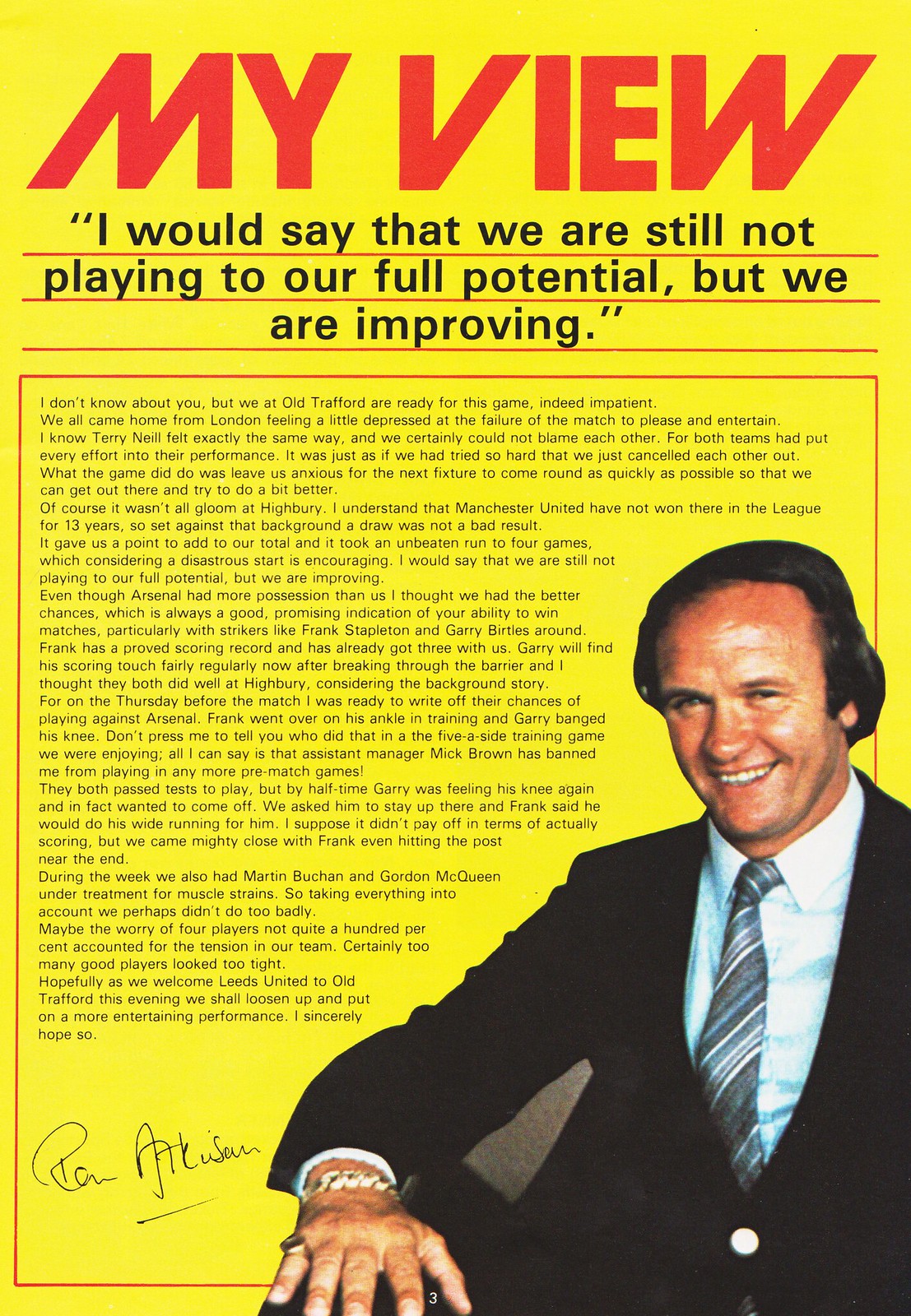This image showcases a magazine page with a bright yellow background prominently displaying a promotional ad or article. At the top, bold red text reads "MY VIEW," spanning the page horizontally. Beneath this title, a quotation in smaller black lettering states, "I would say that we are still not playing to our full potential, but we are improving." The main body of the text is enclosed within a yellow box outlined by a thin red border, filled with several paragraphs of small black type.

In the bottom right corner of the page is a photograph of an older gentleman, smiling while dressed in a sharp black suit. He is wearing a light-colored shirt, possibly white or light blue, and a tie with blue, gray, and white diagonal stripes. Notably, he has a gold ring on the pinky of his right hand and a gold bracelet on his right wrist. His black hair is neatly combed over. Below the text box, the man’s signature is visible, presumably indicating he is the author of the quoted statement and the article. Additionally, the page number "3" is centered at the very bottom of the page.